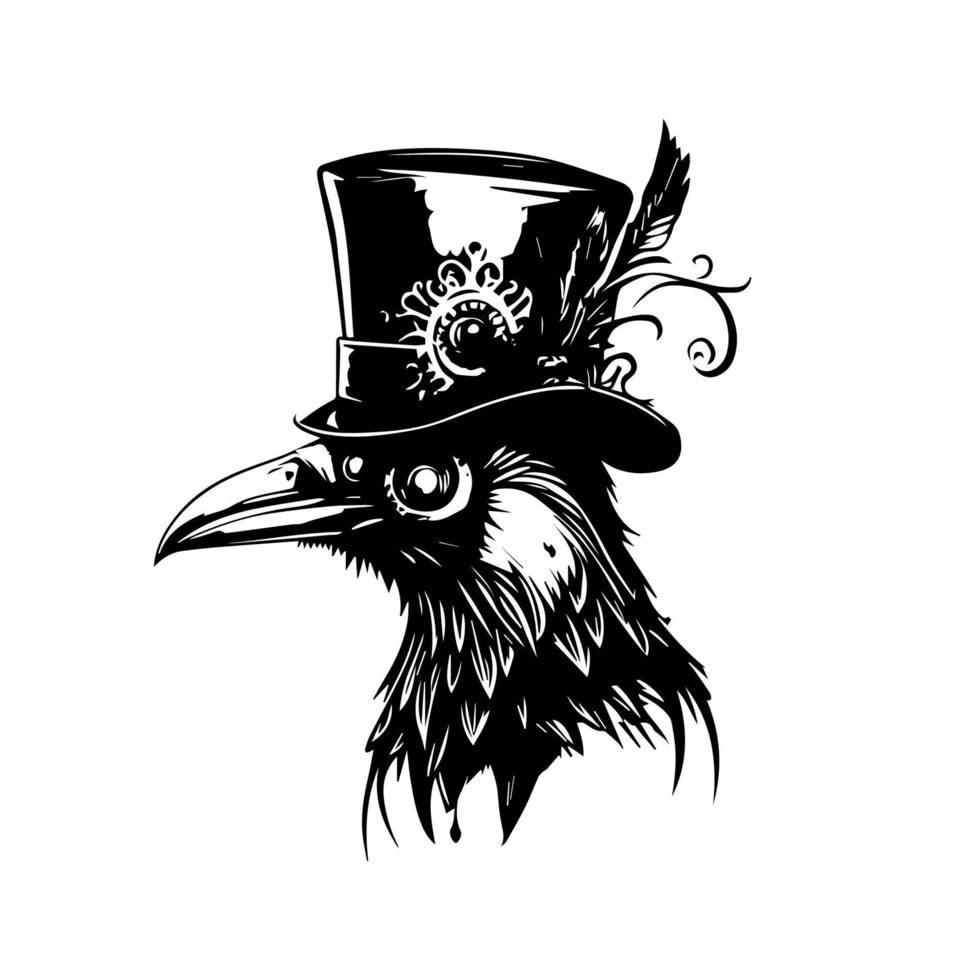This black-and-white drawing depicts a bird, specifically a black bird, featured prominently in the center of the image. The bird is facing left, with its body cut off at the shoulders, revealing only its neck and head. A significant feature of the bird is its large black eye with a white pupil. Adding an enigmatic touch, the bird wears a tall, square-shaped top hat, reminiscent of the style worn by President Lincoln. The hat, which sits snugly atop the bird's head, features a band with an ornate buckle and a decorative feather extending to the right. The brim of the hat has a slight curvature, adding a unique flair. The background is stark white, which highlights the intricate, flowing feathers of the bird and the detailed design of the hat, making the drawing both peculiar and captivating.